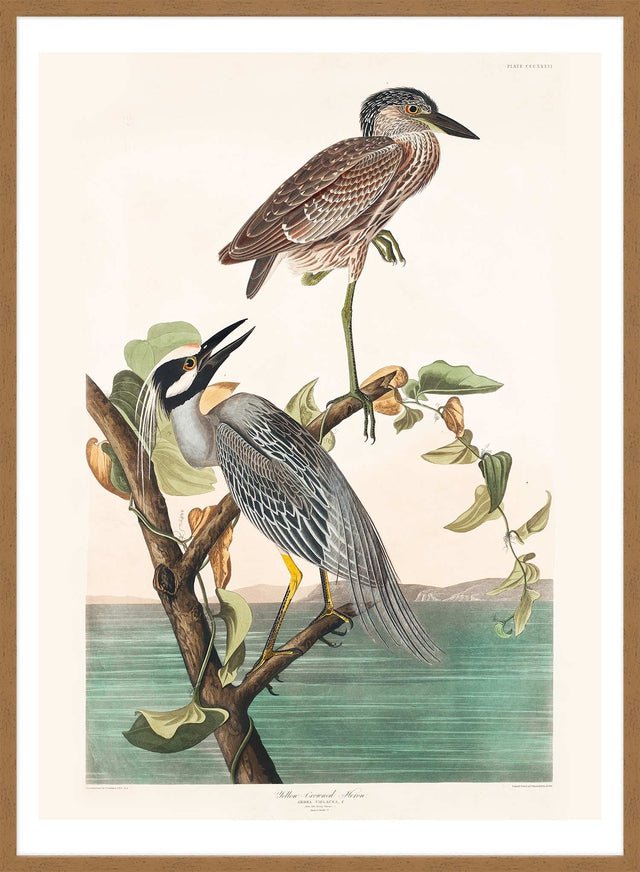This detailed painting, entitled "Yellow-Crowned Night Heron" by John James Audubon from the late 1800s, features a pair of herons perched on a tree limb against an oceanic backdrop. Encased in a thin, medium-tone wooden frame approximately 8 by 10 in size, the artwork is accentuated by a white border framing beige-colored paper. 

The background exhibits a smooth, aqua-blue ocean with greenish hues, capped by gray mountains or hills on the horizon beneath a light pinkish-orange sky. In the mid-ground, a branch adorned with green and brown leaves stretches upward, providing perches for the two herons.

The larger heron in the foreground, identified as a Yellow-Crowned Night Heron, is dark gray with black and white facial markings. Its defining features include long white feathers flowing from the top of its head down its neck, a black beak, and golden legs clutching the limb. This bird gazes upward toward the top-right corner with its neck slightly arched. 

Perched above is a smaller heron with predominantly brown feathers, a black head, and a black beak. This heron also has long green legs and is captured balancing on one leg. It is in profile, facing right, bringing a sense of balance and harmony to the composition.